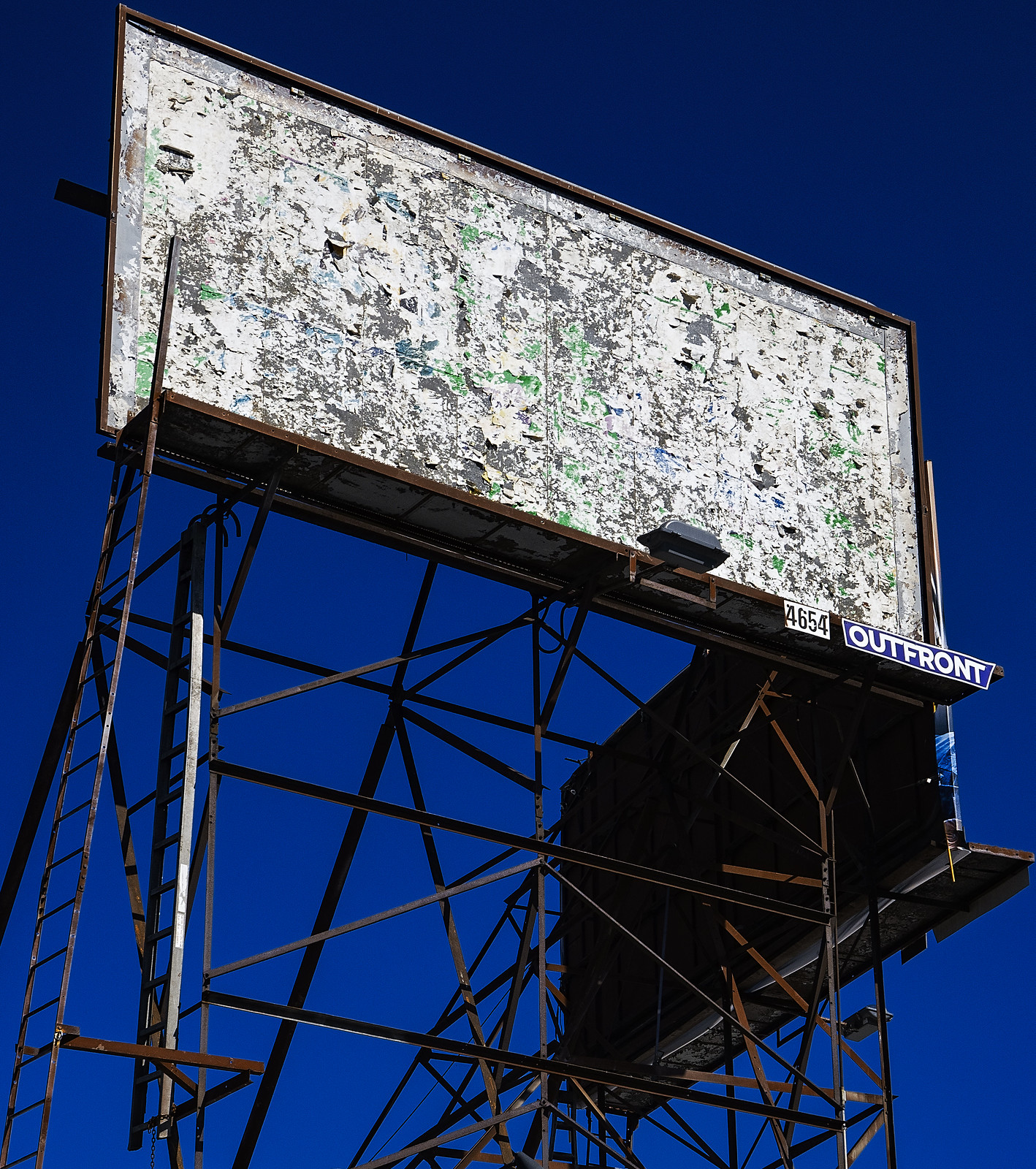The image depicts a well-worn billboard with a predominantly blue background, noticeably faded with time. The center of the billboard features a large white section marred with numerous scratch marks, adding to its weathered appearance. Prominently displayed in white text on the front are the numbers "4654." A ladder is situated on the left side of the billboard, which is supported by rusted metal legs. The sky in the background is a deep, dark blue, contrasting with the colorful array of wear and tear on the billboard itself, including gray, white, green, and brown marks. The overall impression is one of a colorful yet heavily deteriorated sign, marked by the passage of time and exposure to the elements.